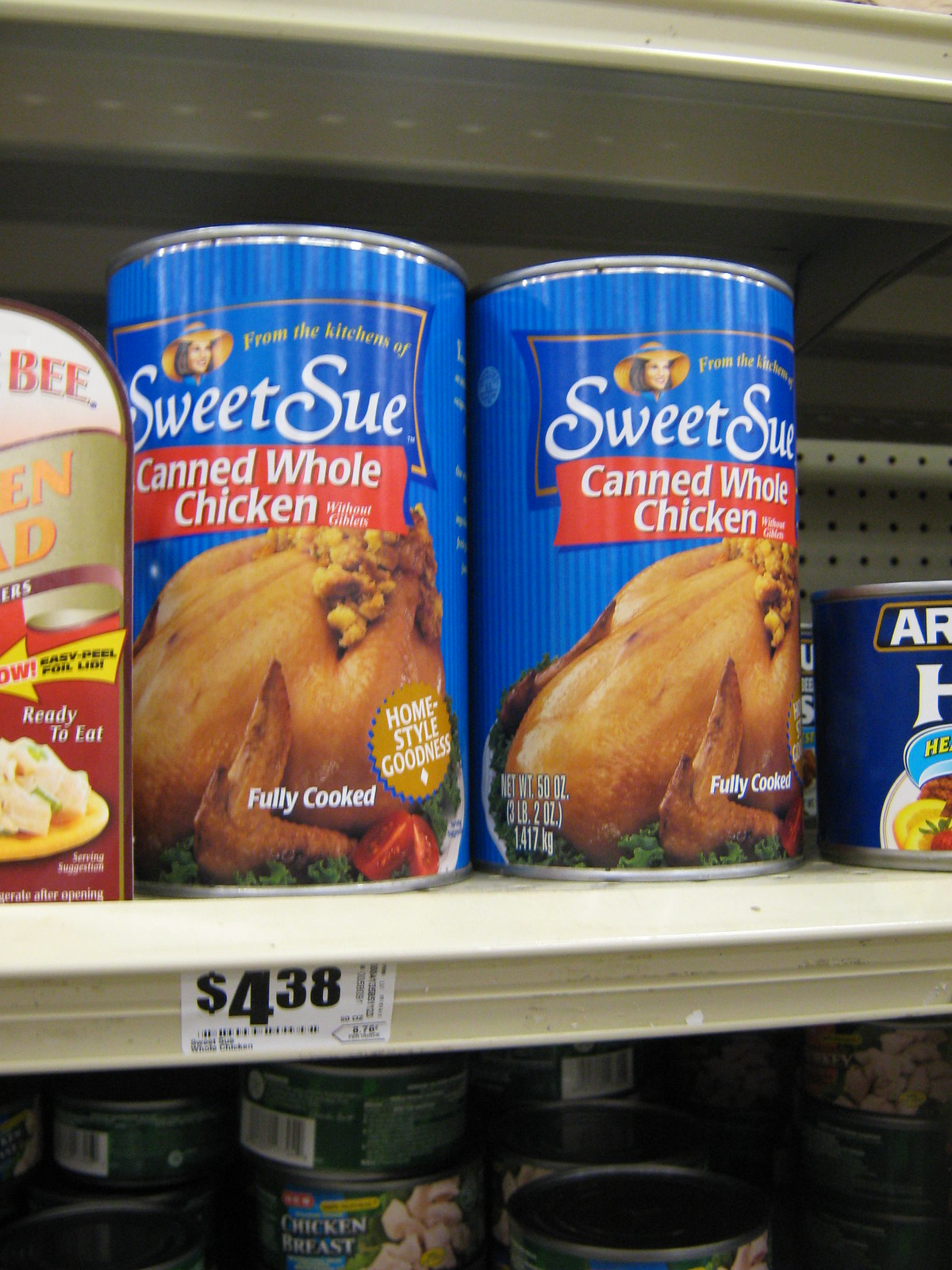This color photograph provides a detailed close-up of a retail shelf at a grocery store, with the shelf itself being a creamy beige color. The shelf features a pegboard design at the back, and we can see perforations from the shelf above. The prominent focus is on the food items displayed on the shelf. On the right-hand side, there are two identical large blue cans, each labeled "Sweet Sue" in white letters, followed by "From the Kitchen of" and "Canned Whole Chicken" outlined in red. The cans display a picture of a whole cooked chicken with garnishing and stuffing. Smaller text indicates the chicken is "Fully Cooked" and offers "Home-Style Goodness." Each can holds 50 ounces, equivalent to three pounds and two ounces. Positioned in front of these cans, on the edge of the shelf, is a white sticker with black printing displaying the price, $4.38. 

On the left-hand side, partially cut off, is a red and white can labeled "B.E.E." in red, with a yellow arrow pointing left, and text indicating "Ready to Eat" with an image of a light-colored dish on a yellow plate. Another can with a blue background and white writing is also partially visible. Above the main shelf, the top of the shelf below is visible, with smaller cans in shadow.